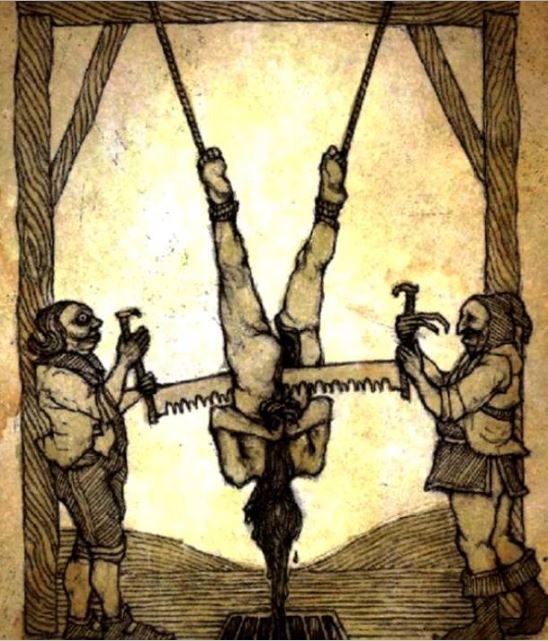This detailed illustration vividly depicts a brutal medieval execution method. The central figure is a nude man suspended upside down by ropes tied to his ankles, which are attached to a wooden arch. His hands are bound behind his back, and his long hair hangs downward. Two men, each dressed in medieval peasant attire with pointy boots and ghoulish faces, stand on either side of him. These men are sawing the victim in half using a large, two-handled saw. The sawing starts from the V of his legs and progresses downward along the spine, slicing through his buttocks and back. Blood streams from the sawing wound, dripping over a metal grate positioned below. The scene has a sepia and brown color palette with black outlines, emphasizing its graphic and historical nature.